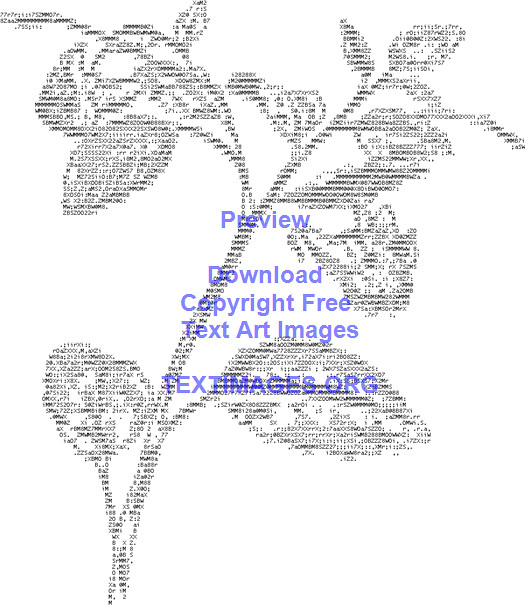The image features a dark gray plant, somewhat resembling a flower that could be a rose, though the specific species is indiscernible due to the blurry, pixelated nature of the image. This pixelation is a result of the intricate design, which is composed entirely of small letters and numbers that form the larger plant shape. The plant has a stem angled at approximately 45 degrees, stretching from the bottom left to the top right, with leaves branching out to the left and right. The background of the image is stark white, providing a sharp contrast to the black plant silhouette. Overlaying the image is a lavender-colored watermark in a sans serif font, stating "Preview download copyright free text art images" and "textimages.org." Additionally, there is some very small, illegible text integrated into the plant design itself. This watermark likely serves to prevent unauthorized use and credit misappropriation of the artwork.